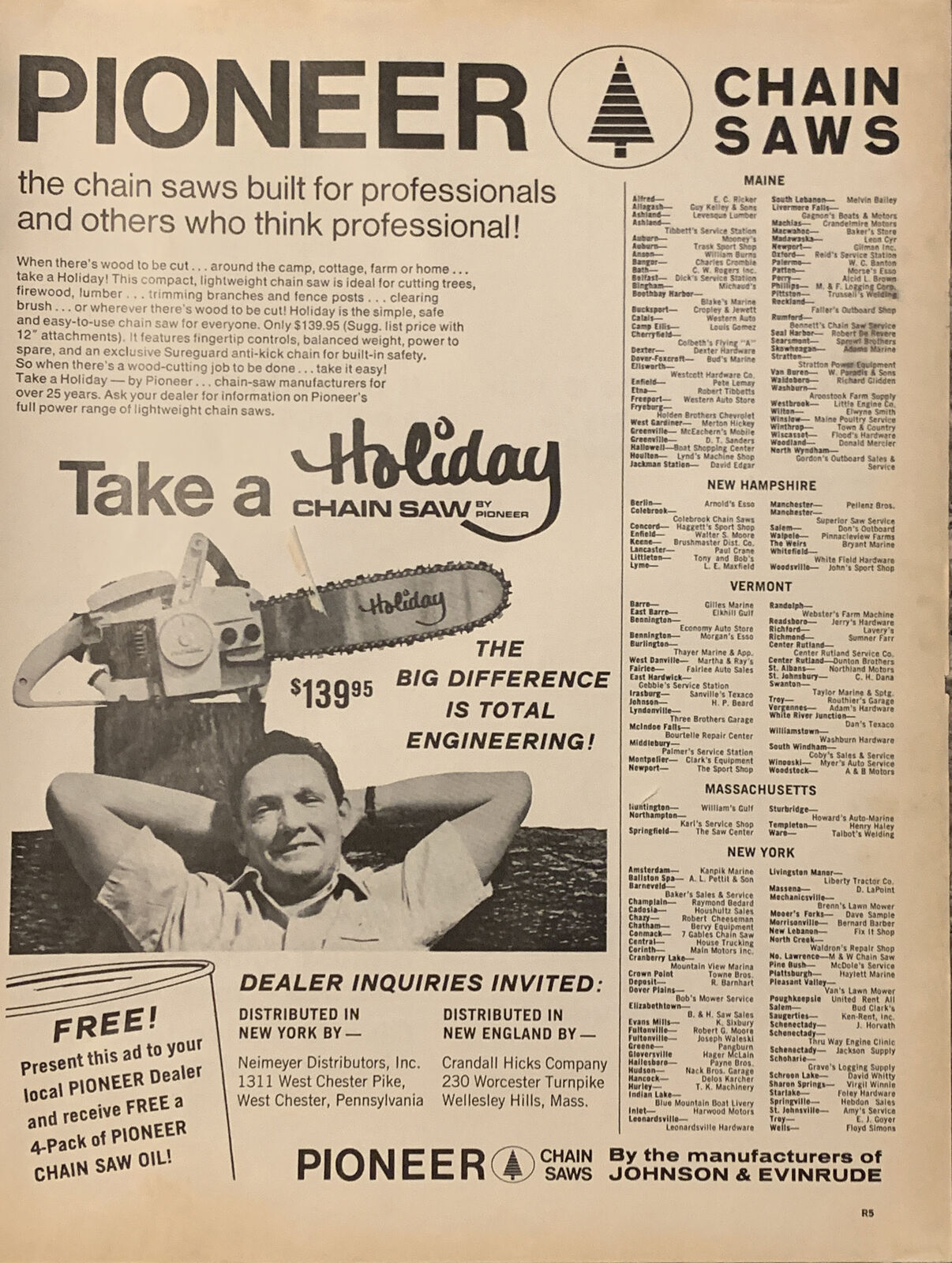This vintage black-and-white advertisement showcases Pioneer Chainsaws, renowned for being "built for professionals and others who think professionally." Prominently displayed at the top is the brand name, flanked by a circular logo featuring a tree. The ad emphasizes the chainsaw's exceptional engineering, stating, "The big difference is total engineering," and features a special promotion: presenting the ad to a local dealer awards a free four-pack of Pioneer Chainsaw Oil. In the image, a relaxed man leans back against a large cut log with his hands behind his head, his trusty chainsaw atop the log, signifying an easy day's work. On the right, there's an extensive list of dealers across Maine, New Hampshire, Vermont, Massachusetts, and New York, with Maine having the longest list. Additional text at the bottom highlights dealer inquiries are invited and mentions distribution specifics for New York and New England. The chainsaw is priced at $139.95 and is produced by the manufacturers of Johnson and Evinrude.